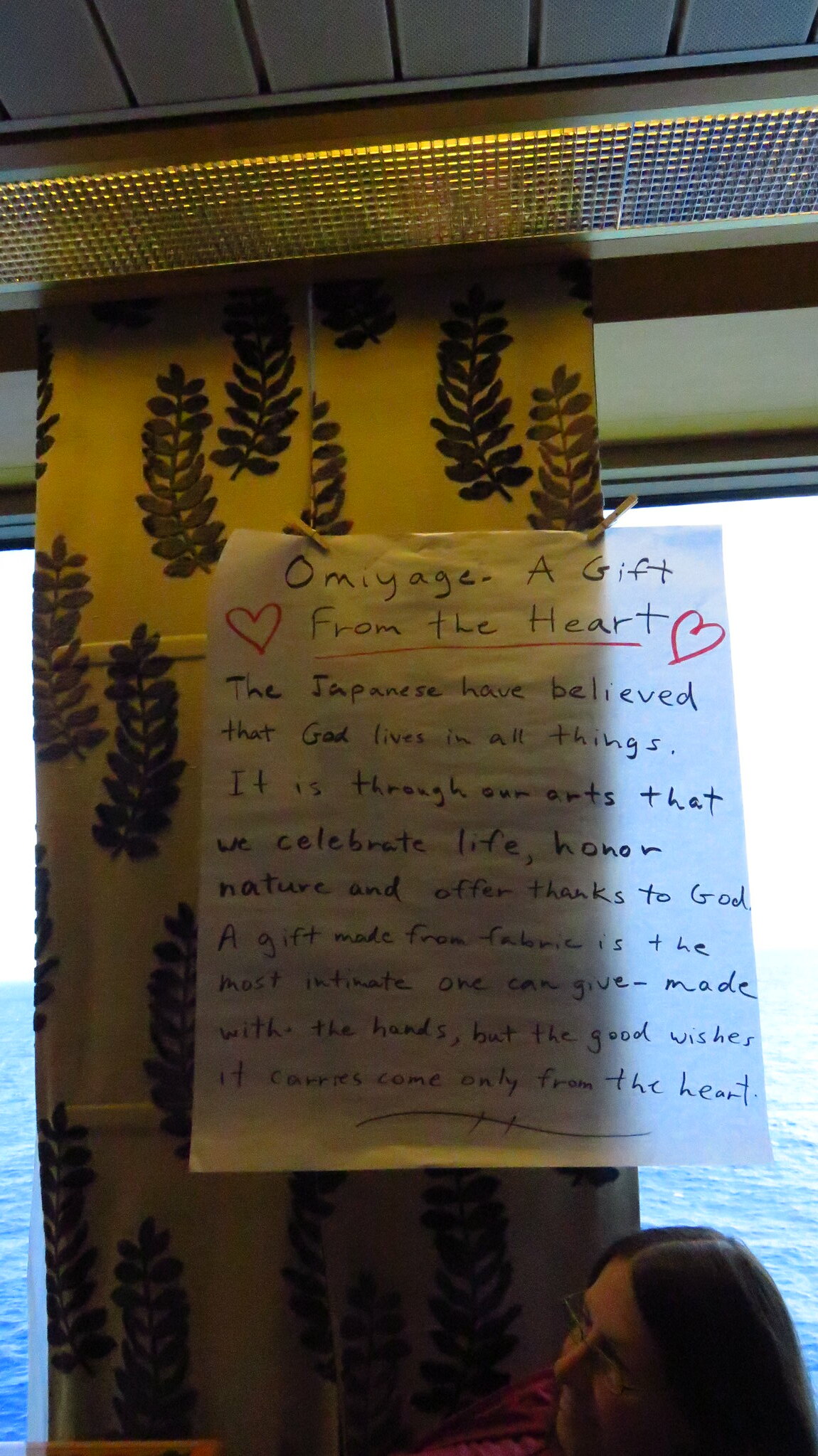The photo features a note, handwritten in black ink on a thin, almost see-through paper, pinned to a beige panel adorned with decorative blue and green vine-like leaves. The panel is set in front of a large glass window, through which water can be seen, suggesting the image might have been taken from a cruise ship. The note is titled "Omiyage, A Gift from the Heart," with the title underlined and flanked by two red hearts. The message on the note reads: "The Japanese have believed that God lives in all things. It is through our art that we celebrate life, honor nature, and offer thanks to God. A gift made from fabric is the most intimate one can give. Made with the hands, but the good wishes it carries come only from the heart." In the bottom right corner of the photo, a woman with long, slightly graying black hair, wearing glasses and a red shirt, is visible in profile, looking towards the left. The entirety of the photographed scene is bathed in light, highlighting the contrast between the note's delicate script and the vibrant, life-infused setting.